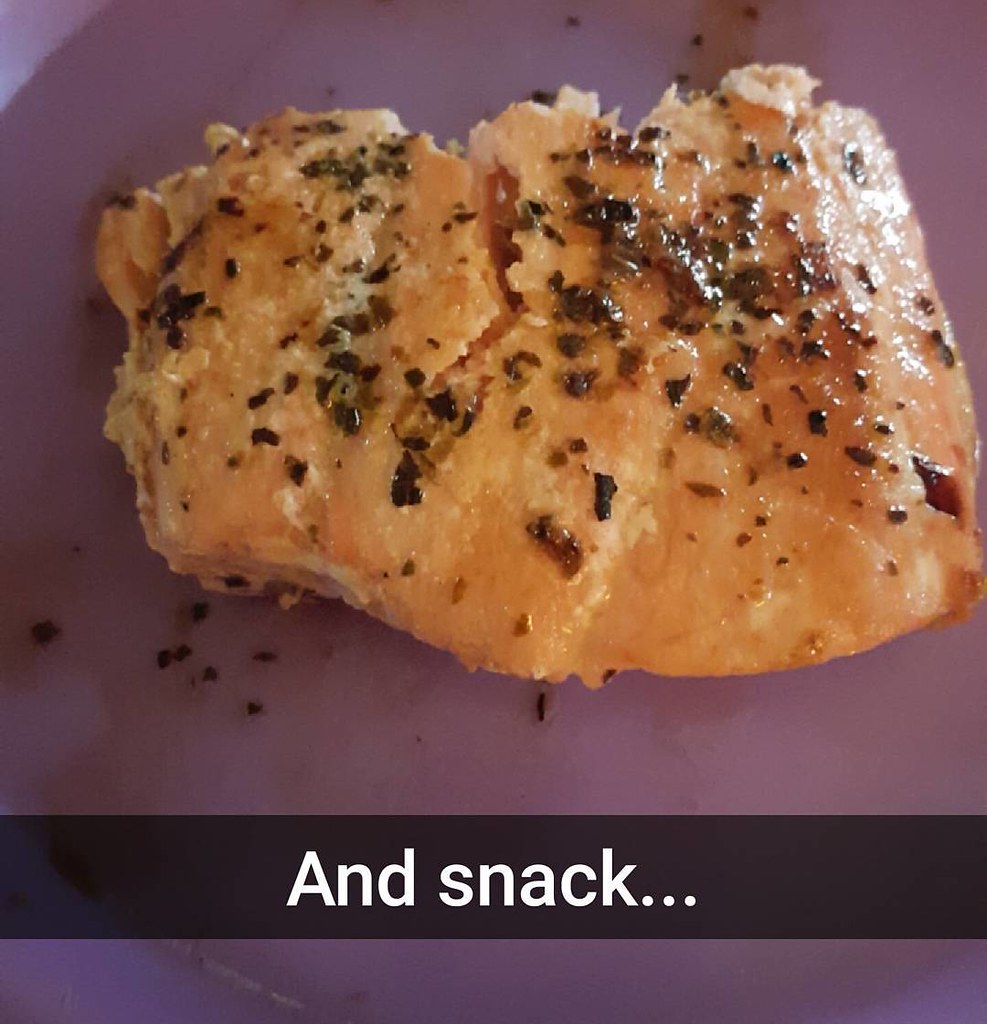The image depicts a small, broken or bitten-off piece of cooked salmon, likely seasoned with various spices, giving it a dark brown and black flecked appearance. The salmon, with a slight crack down the middle, sits on a light-colored, possibly pink or purple, plate or bowl with an oily glaze, which reflects a bit of light. Despite some ambiguity from the shadows and reflections, the main focus is on the seasoned, glossy salmon, which occupies most of the frame. Underneath the food, a dark, semi-transparent bar spans the bottom of the image with the white text "and snack..." written in a style reminiscent of a Snapchat overlay.